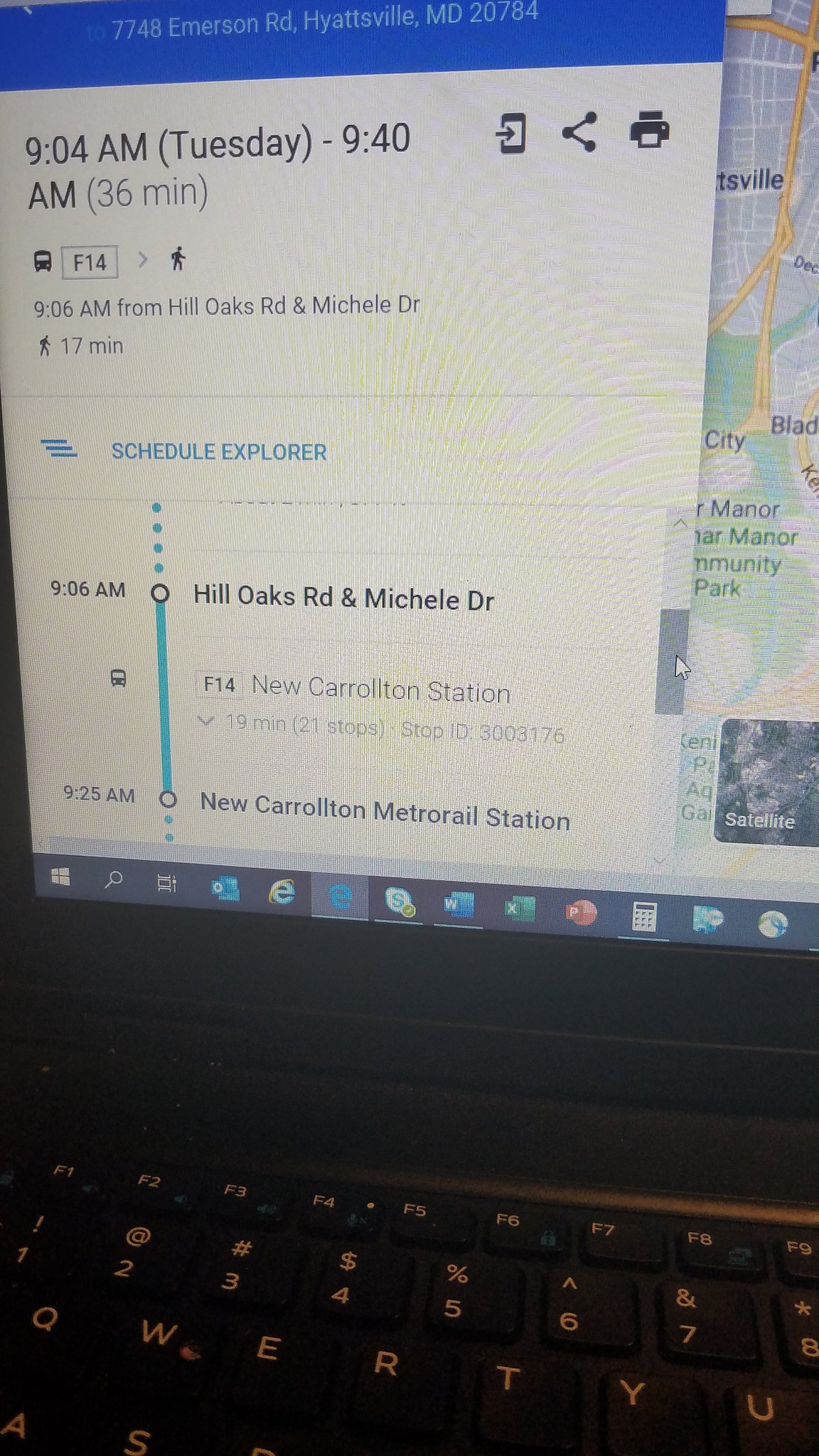The image depicts a computer laptop with its keyboard prominently displayed. On the screen, a detailed digital display interface is visible. At the top of the screen, the text reads "7748 Emerson Road, Hyattsville, MD, 2074." Further down, there’s a timestamp that says "9:04 AM (Tuesday) – 9:40 AM." The display also includes a cellphone icon with an arrow pointing towards it, followed by a series of dots connected by lines, and a printer icon.

Below that, there's additional text which reads "9:06 AM from Hill Oaks Road and Mitchell Drive." This is followed by symbols indicating different modes of transportation: a bus with the label "F14" and an arrow pointing to a walking person. It further states "72 minutes (schedule - 4)."

On the left side of the display, another schedule is shown as: "9:06 AM" with an arrow pointing down to "9:25 AM." At the top of this section, it again mentions "Hill Oaks Road and Mitchell Drive." The line below this says "F14 to New Carrollton Station" and beneath that, "New Carrollton Metro Rail Station."

In summary, the image captures a complex and detailed transportation schedule interface displayed on a laptop screen, complete with addresses, timestamps, transportation modes, and route information.